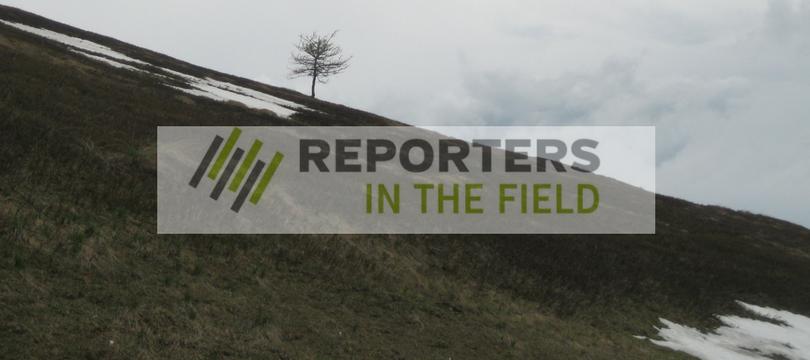The image depicts a green-brown hillside field, angled from the top left to the bottom right, strewn with patches of snow indicating an early winter or spring setting. A solitary bare tree stands towards the top left, framed by a cloudy, gray sky with varying shades of darker clouds. Superimposed in the middle of the image is a white rectangular poster. It displays the words "REPORTERS" in black all-caps font and "IN THE FIELD" in green all-caps font. To the left of the text, six diagonal lines—three green and three black—slant from top right to bottom left, forming a part of the logo.